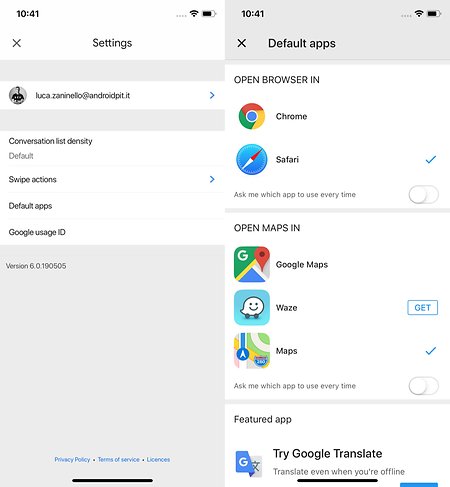### Detailed Caption:

The image showcases two different screens side by side, both displaying user interface elements from a mobile device, likely running on an Android operating system.

**Left Screen:**

- **Current Time Display:** 
  - The screen shows "10:41" in black text.
- **Settings Menu Overview:** 
  - A partially colored battery icon indicating roughly 75% charge.
  - A volume icon.
  - A gray banner beneath these icons.
- **User Profile and Email:** 
  - A black-and-white profile picture of a user named Luca Zanilio.
  - The associated email: "lucazanilio@android.it.it".
- **Settings Sections:**
  - "Conversation list density" with a blue arrow pointing to the right, indicating a navigable option.
  - "Swipe actions" also accompanied by a blue arrow pointing to the right.
  - "Default apps" and "Google usage ID."
- **Version Information:**
  - Text in gray: "Version 6.0-190-505."
- **Legal Links:** 
  - At the bottom, clickable blue text links for "Privacy Policy," "Terms of Service," and "Licenses."

**Right Screen:**

- **Current Time Display:** 
  - The screen shows "10:41."
- **Default Apps Menu:**
  - The title "Default apps" is displayed in black with an "X" on the left for closing the menu.
  - Standard icons for signal strength and battery status are visible.
- **Browser Selection:** 
  - Header: "Open browser in."
  - Options to choose between Chrome (icon in red, green, yellow with a blue center) and Safari (icon with a blue compass and red/yellow hands).
  - Safari is selected, indicated by a blue check mark.
  - A toggle switch under "Ask me which app to use every time" which is turned off (gray and white).
- **Maps Application Selection:**
  - Header: "Open maps in."
  - Options include Google Maps (G icon with a red location pin) and Waze (blue square with a white ghost icon).
  - Google Maps is selected, indicated by a blue check mark.
  - Another toggle switch under "Ask me which app to use every time" which is again turned off (gray and white).
- **Additional Features:** 
  - A featured section suggesting "Try Google Translate," with the message "Translate even when you're offline," and displaying the Google Translate icon.

The detailed settings and the visual representation of icons and toggles provide an insightful look at device customization options, reflecting user preferences for default applications and user experience settings.